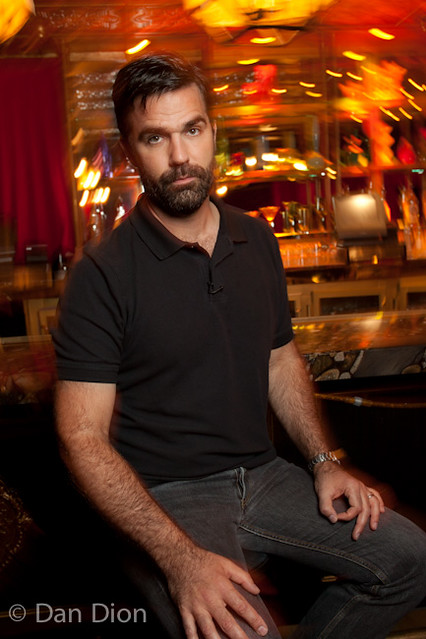This color photograph, attributed to Dan Deon, features a man likely in his mid-30s, sitting on a stool and posing for a profile picture, possibly for a website. The man has short dark brown hair, a full dark brown beard, and is looking directly at the camera with his calm, brown eyes. He wears a black collared shirt with short sleeves, paired with black denim jeans. His left wrist sports a watch, and his noticeably hairy arms add a distinct feature to his appearance. The background, a bar setting blurred intentionally to create a depth of field effect, showcases spinning lights and an orange hue, adding a dynamic and vibrant feel to the image. The colors blend together, hinting at motion distortion, which contrasts with the man's clear and composed presence. A subtle watermark on the bottom left corner reads "Dan Deon," signaling the photographer’s credit.